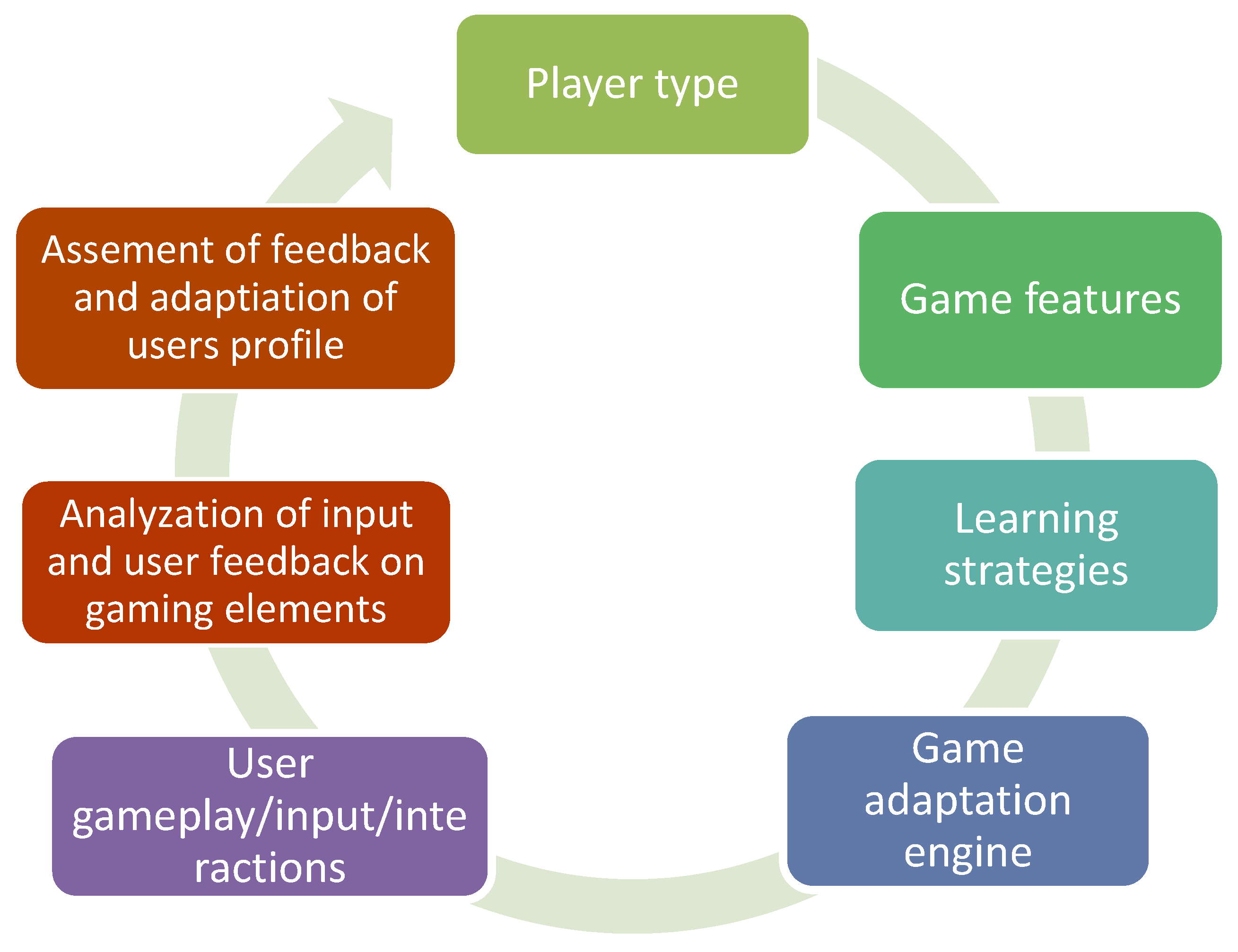This image showcases a circular flowchart composed of small, rectangular, brightly colored boxes with a pale green circle in the background interconnecting them. The flowchart begins at the top with a box labeled "Player Type," and continues sequentially with boxes titled "Game Features," "Learning Strategies," "Game Adaptation Engine," "User Gameplay/Input/Interactions," "Analysis of Input/User Feedback on Gaming Elements," and "Assessment of Feedback and Adaptation of User Profile," looping back to "Player Type" to complete the circle. The boxes transition through a gradient of colors from shades of green, to blue, to purple, and finally to a burgundy hue. Each box contains white lettering, creating a vibrant, visually appealing diagram that effectively illustrates the cyclical nature of player interaction and game adaptation feedback.